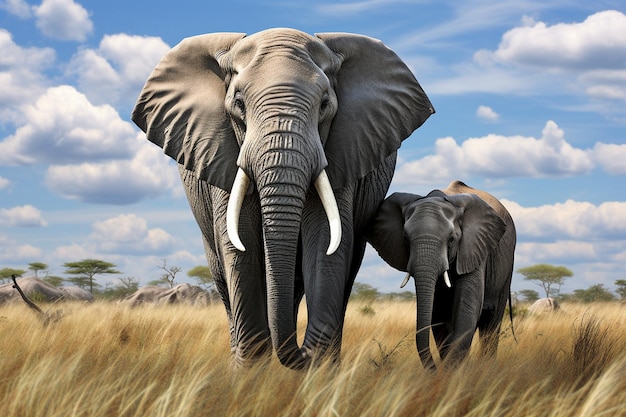A highly detailed and possibly AI-generated image showcases two elephants, a large adult and a smaller juvenile, walking towards the viewer on the African plains. The adult elephant, with strikingly white tusks, exhibits a textured gray skin so detailed you can almost count the ridges. To its right, the young elephant, about half the size of the adult, has smaller tusks and mimics the adult's forward gaze. They traverse through tan or beige savannah grass. The backdrop features a brilliantly clear, expansive blue sky adorned with fluffy white clouds, accentuating the crisp, almost surreal quality of the image. Sporadically, small and varied savannah trees dot the horizon, contributing to the natural, yet slightly edited feel of the scene. The landscape is devoid of other animals, emphasizing the bond and parent-child relationship between the two elephants as they journey across the pristine terrain.